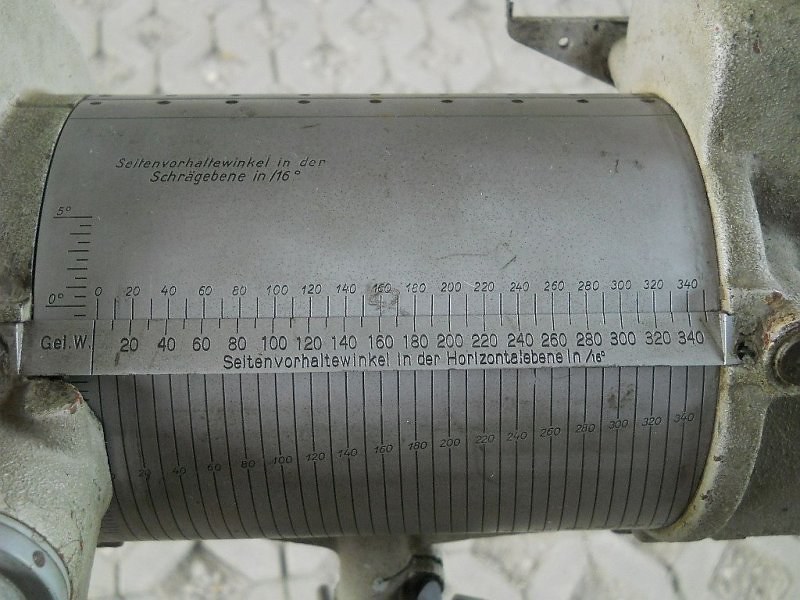The image features a close-up of a cylindrical metal mechanism, possibly a pipe, set against a light white-grayish background. The pipe bears various markings, including a measurement system with tiny tick marks and numerical values increasing from zero in increments of 20, reaching up to 340. Numerous pieces of text in German, along with numerical values likely indicating angles or other measurements, are displayed prominently across the pipe. In the middle left-hand corner, the text "gel w" can be observed. Toward the right side of the image, a rusted or stone-like clamp tightly secures the pipe. The top of the pipe showcases nine indents, where rivets or screws seem to be fastened. Extending from the bottom of the pipe is a smaller pipe that descends into what appears to be the ground or another surface area.